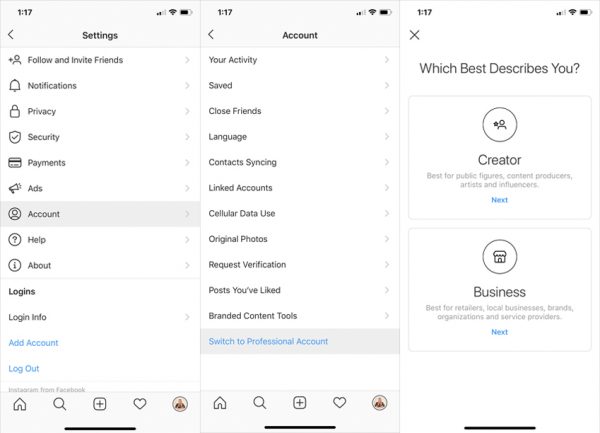The image displays a mobile device's screen, divided into three columns. Each column represents a separate page. Focusing on the first column to the left:

- **Top Bar Details:** 
  - **Time Display:** "1:17" is shown in the upper left corner.
  - **Signal Strength:** To the right of the time, there are four bars indicating signal strength, with the first two bars in black and the last two in gray.
  - **Wi-Fi Indicator:** A fan-like icon, likely representing Wi-Fi connectivity.
  - **Battery Status:** The battery icon shows that the device is mostly charged, depicted in black.

- **Main Section:**
  - **Navigation and Header:**
    - **Back Arrow:** A left-pointing arrow that reads "Settings."
    - **Current Section:** Labelled as "Bulb Base," written in black type.
  
  - **Options Menu:**
    - **Invite Friends:** An icon of a person with a plus sign, with the text "Follow and Invite Friends" to its right, followed by a right-pointing arrow in gray.
    - **Notifications:** A bell icon with "Notifications" text, accompanied by a right-pointing arrow.
    - **Privacy:** A lock icon labelled "Privacy," also with a right-pointing arrow.
    - **Security:** A shield with a checkmark, captioned "Security," with a right-pointing arrow.
    - **Payments:** An icon of a credit card next to the text "Payments," followed by a right-pointing arrow.
    - **Ads:** A bullhorn icon with the text "Ads," and a right-pointing arrow.
    - **Account:** A grayed-out person icon with the text "Account," followed by a right-pointing arrow.

The detailed description ensures a clear understanding of each element present in the first column of the displayed mobile device screen.